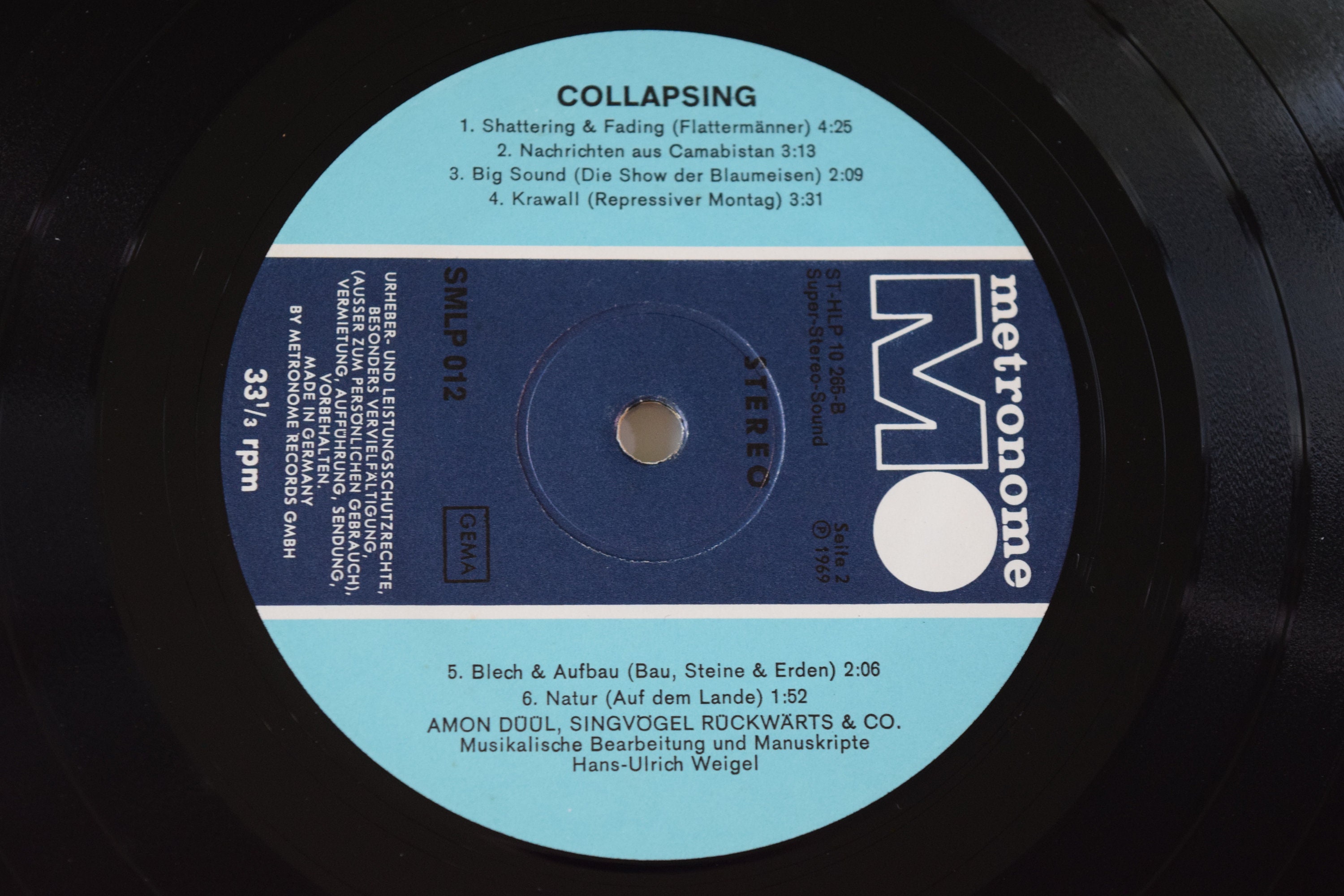This image captures the center label of a 33⅓ RPM vinyl record by Metronome Records. The label is presented in a rectangular picture, focusing tightly on the central portion and slightly extending to the black trim where the needle is placed. The design features a horizontal striped pattern: light blue at the top, followed by a white stripe, then a dark blue section in the middle, another white stripe, and light blue at the bottom. At the top, in black text, is the album’s name, "Collapsing," with a list of six songs in the light blue sections. The dark blue stripe prominently displays "Metronome MO" in white writing, along with a large "M" emblem and additional lettering. The record seems to come from a European company, possibly Germany or Amsterdam, as indicated by mentions of "Amon, Dual, Singvogel, Rockworts and Company" in the light blue area. Each song appears to be around four to five minutes long, making a total playtime of approximately 20 minutes.